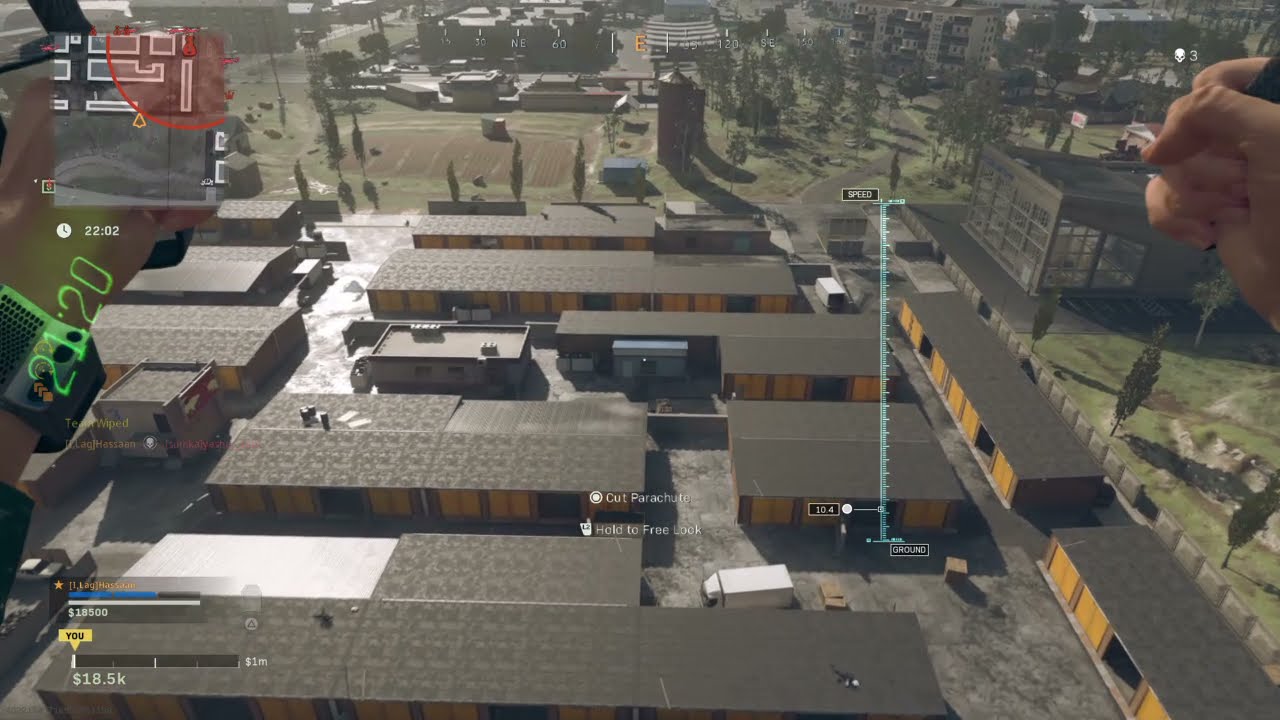The image depicts an aerial view of a post-apocalyptic video game scene set in a gloomy, run-down environment. The main focus is on a series of long, low, yellow-walled storage units with gray roofs, situated in an industrial complex. Scattered around are various buildings of different shapes, some clustered along a fence line and others in open areas. A solitary white van is parked in front of one storage building. Off in the distance, there's a town, tall multi-story buildings, and what appears to be a sports field with marked ten-yard lines, as well as several silos. The bottom left corner of the image displays a point system with a money line marked 2120, and an upper left corner shows a mini-map indicating the player's location. Greenery and trees are visible towards the upper part of the image, emphasizing the desolate yet sprawling environment. Visible in the foreground are two hands; one on the right is gripping something, possibly indicating a VR perspective, and the other in the upper right corner is balled into a fist with the fingers and thumb visible, facing the viewer.